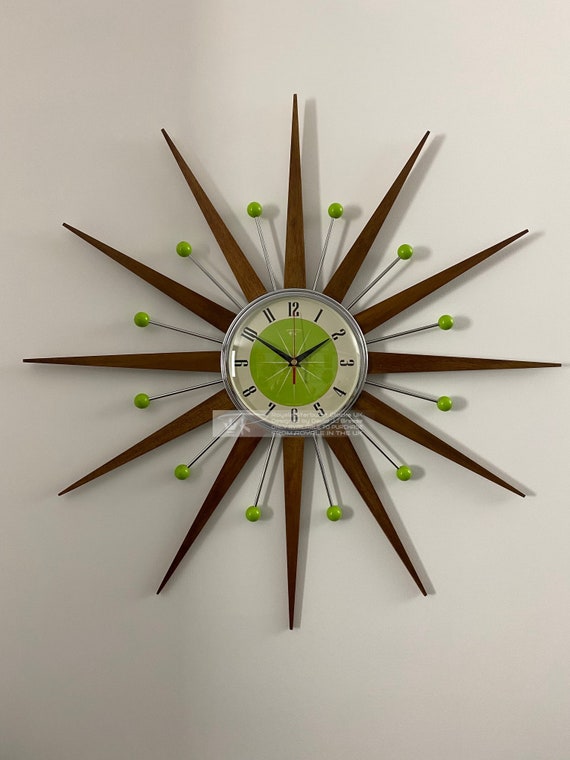This is a rectangular-shaped image with a beige background that features a sophisticated, art-like clock, taller than it is wide. The clock, hanging on a plain wall, resembles a starburst with long, brown triangular prisms radiating outward. Between each brown prism, there is a wire ending in a small green ball, akin to sewing pins. The central part of the clock is a metal circle enclosing a beige face with black numbers from 1 to 12. Inside this beige circle is an additional lime green circle where the clock’s hands point to 10:10 or 1:50. The clock not only tells the time but also stands as a decorative art piece.